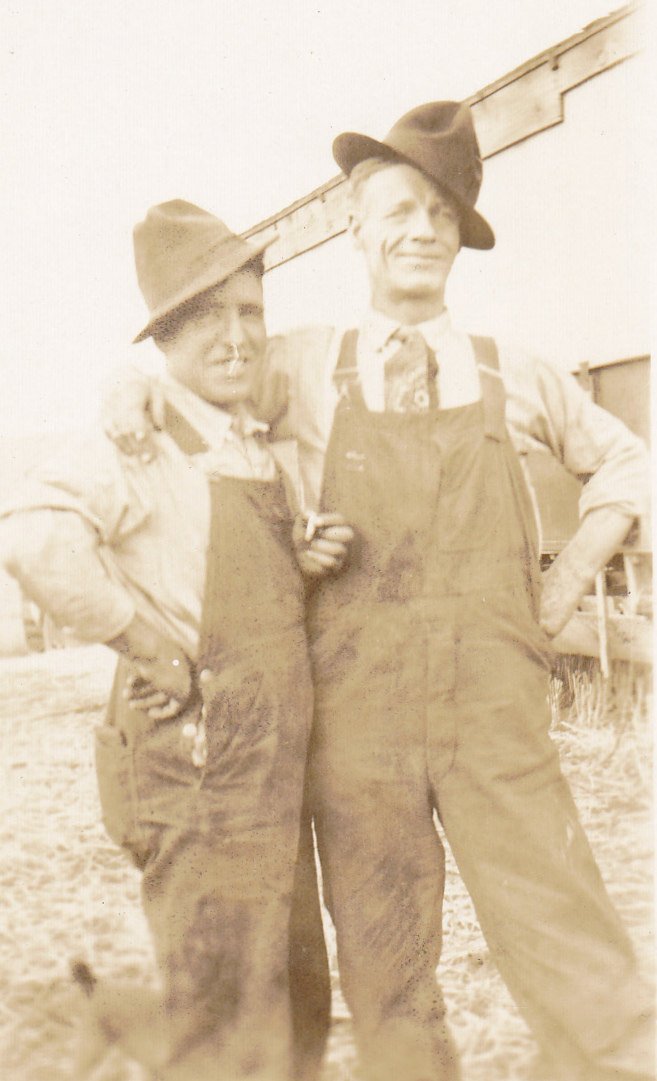The sepia-toned portrait depicts two fair-skinned men in a rustic, possibly early 20th-century setting, a detail emphasized by the weathered, partially damaged edges of the photograph. Both men, dressed in overalls and dress shirts with ties, exhibit a relaxed camaraderie, each donning hats jauntily cocked to opposite sides— the man on the left to the left, and the man on the right to the right. The shorter man on the left, sporting dirty overalls with one button unfastened, stands sideways with his right arm on his hip, and his left arm between them. His taller companion on the right, characterized by a thin frame and light-colored eyes, mirrors the relaxed posture with his right arm affectionately draped over the shorter man's shoulder and his left arm cocked similarly. Both men smile, looking directly at the camera, exuding warmth and familiarity. Behind them, a blurred, indistinct large structure, possibly a barn, suggests a farm setting, with hints of animals and a small dog at the shorter man's feet, adding to the rural tableau.